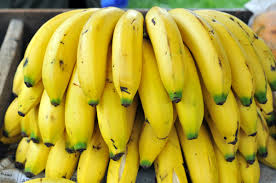This image captures a large bunch of bright yellow bananas, meticulously arranged in three distinct rows with approximately 10-12 bananas per row. The cluster, captured from the bottom angles, reveals the bananas' slightly green tips and black blemishes scattered across their peels. Two bananas in the lowest row have split open, exposing the white flesh within. Dominating nearly the entire frame, the bananas appear ready to be eaten and could belong in a grocery store display. The slightly blurred background suggests the photo is taken outdoors, featuring a green grassy area, a wooden bench or crate, and possibly a faint glimpse of a face in the top right corner. The negligible background detail emphasizes the vibrant, abundant pile of bananas, highlighting their readiness for consumption.